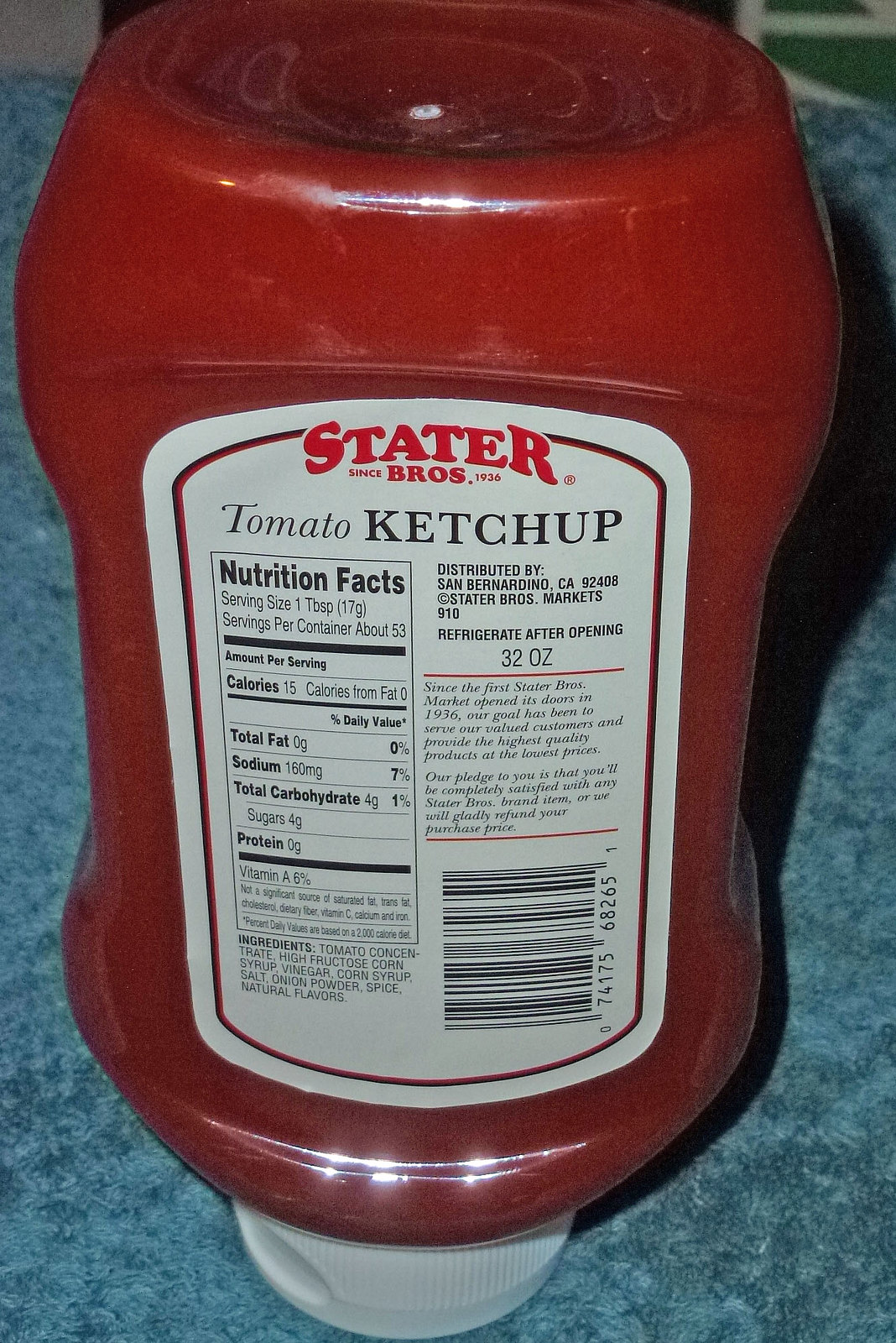The photograph showcases the back of a typical bright red ketchup bottle positioned lid-down on a stylish blue marbled countertop. The marbling on the countertop features a mix of turquoise light blue and gray hues, creating a modern and clean backdrop for the red bottle. The bottle itself has a white lid and retains the classic shape commonly associated with tomato ketchup containers.

The bottle's label is rectangular with rounded edges, giving it a polished look. At the top of the label, you can see "Stater Bros" printed in a bold red font, followed by "Tomato Ketchup" in a black font. The left-hand side of the label prominently features a Nutrition Facts box and a comprehensive list of ingredients. Meanwhile, the right-hand side provides information about the company. Completing the label at the bottom is a standard black and white barcode.